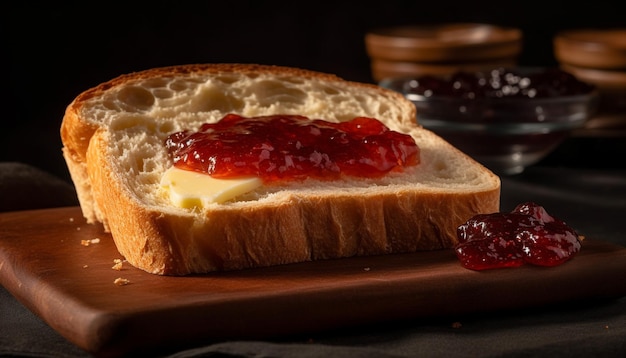The photograph showcases a large, homemade slice of bread centrally positioned on a brown wooden cutting board. The bread is topped with yellow butter and a layer of red jelly, which appears to have seeds, suggesting it could be raspberry jam. Some jelly has slid off and rests on the cutting board in front of the bread. A portion of the cutting board is adorned with additional items, including a container of what seems to be blackberries or a darker jam, and this container is located behind the bread. In the background, blurred brown mugs and additional bowls can be seen, creating a rustic and homely scene. The overall lighting is dark, with a warm, yellowish light illuminating the bread and its toppings, highlighting the textures and colors vividly.